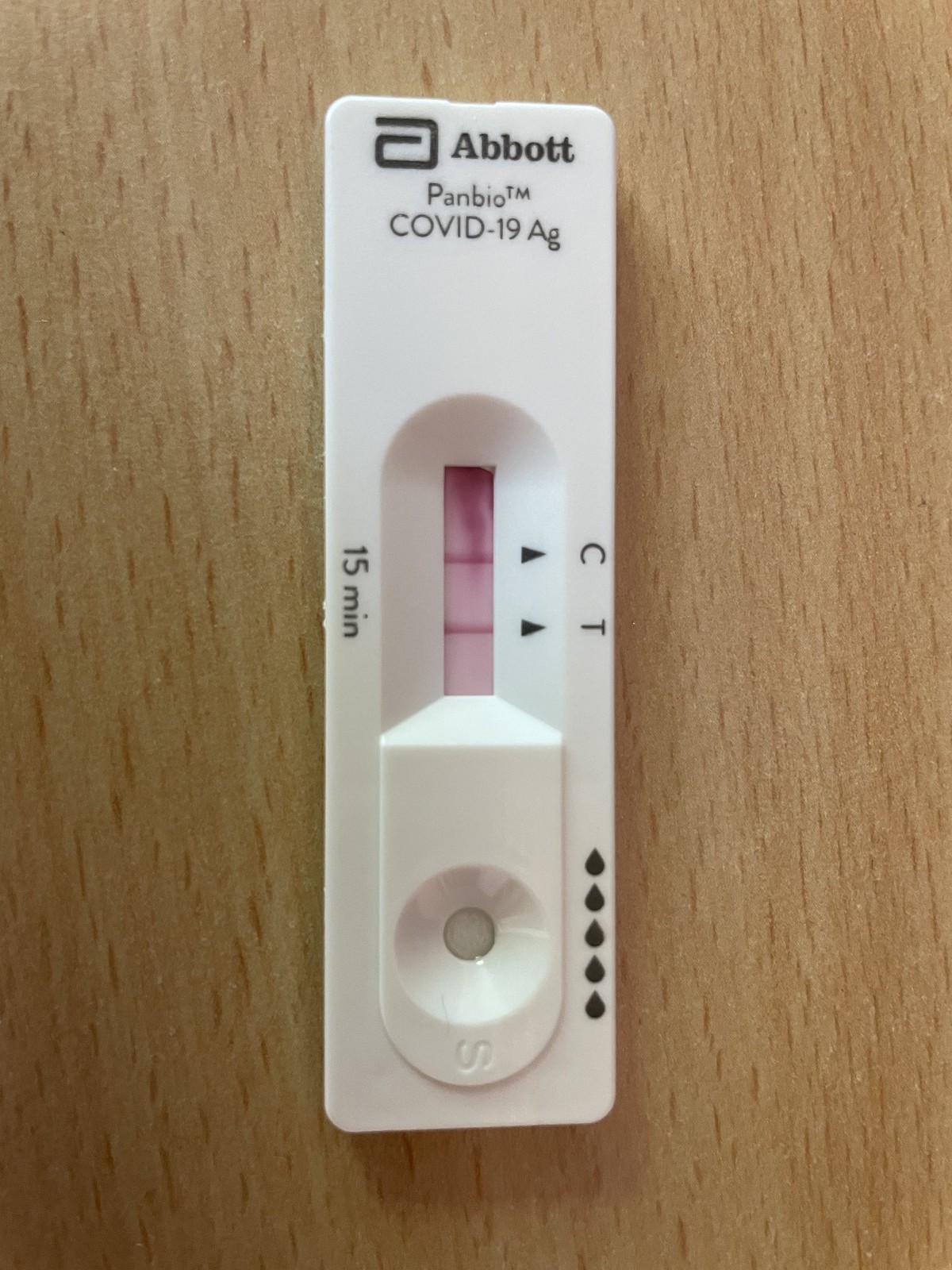Photograph of a COVID-19 test device from Abbott Laboratories. The device, identified as a PanBio™ COVID-19 AG Rapid Test, features a trademarked PanBio label with a prominent "AG" denoting antigen testing. The test has a small window displaying two lines, with arrows pointing to the letters "C" (control) and "T" (test). This indicates that the results are read based on the line positions. The test promises results within 15 minutes. Another noticeable feature is an indentation potentially designated for placing a drop of blood or sample. The plastic device is placed atop a light blonde-colored wooden table, offering a contrast that highlights its functional details.